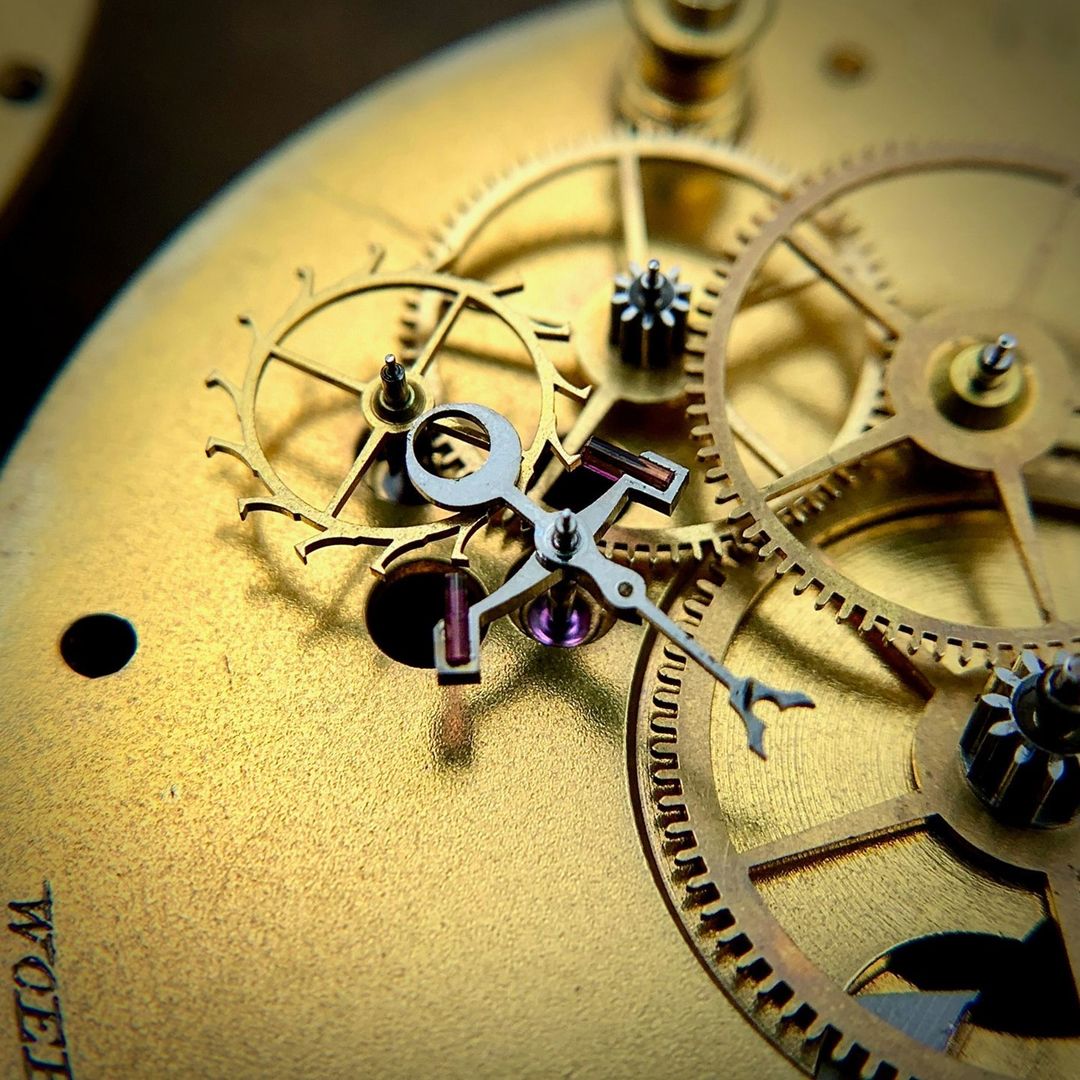The image is a high-quality, close-up photograph of the intricate inner workings of a watch, showcasing a complex and delicate arrangement of gears and mechanisms. The perspective is approximately square, highlighting the precise, even dimensions. The gears are set against a golden metal plate with a mix of bronze, copper, and black-toned cogs, varying in size and shape. Some gears have traditional teeth, while others feature unique, elongated edges designed for specific timing functions. A prominent metal arm, resembling a stick figure with multiple hammers, is positioned above and interacts with the gears to facilitate their movement. Additionally, the surface features fragmented lettering spelling "W-O-E," although it is cut off and incomplete. This detailed assemblage reflects the precision and craftsmanship typical of fine watchmaking.